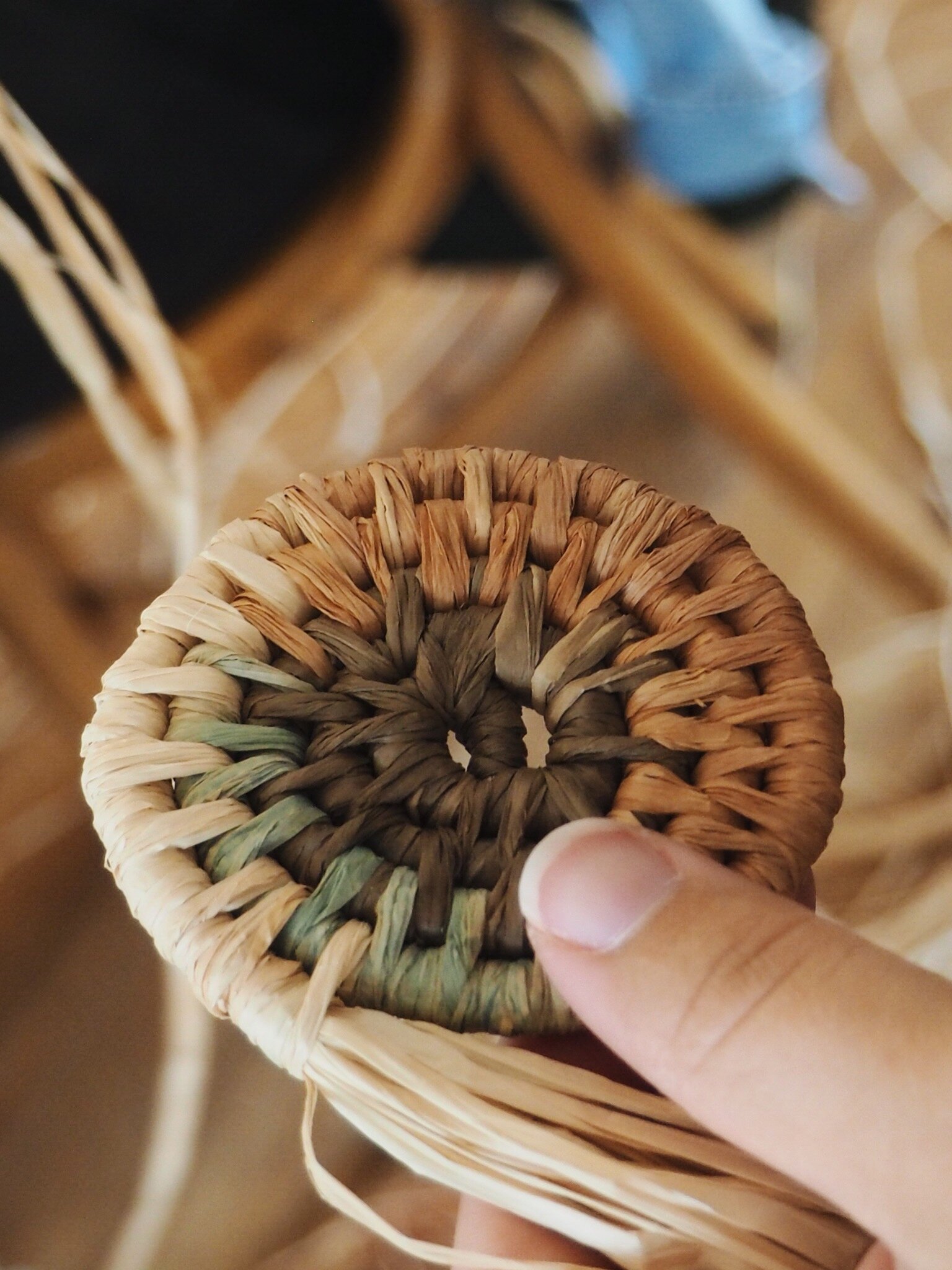In a vertically aligned rectangular picture, a young lady's left hand is prominently featured holding a finely crafted, intricate wicker item. Her thumb, complete with a visible nail, grips the top of this round, woven piece, though her other fingers are out of sight. The skillfully woven object showcases multiple shades of brown, transitioning from medium brown on one side to light brown on the other, with a dark brown center. Adding to the complexity, there's a blend of greenish and reddish weaves amidst the pattern, and the bottom edge of the item has tassel-like extensions. The background is a blur of similar wicker or straw materials in various brown tones, blending seamlessly and creating an indistinct backdrop. A solid black area occupies the upper left corner, while light enters the frame from the right, illuminating parts of the scene. Beneath the wicker object, out-of-focus details suggest it rests partially on what appears to be a wooden floor, and a similarly woven chair is situated at the top of the image.